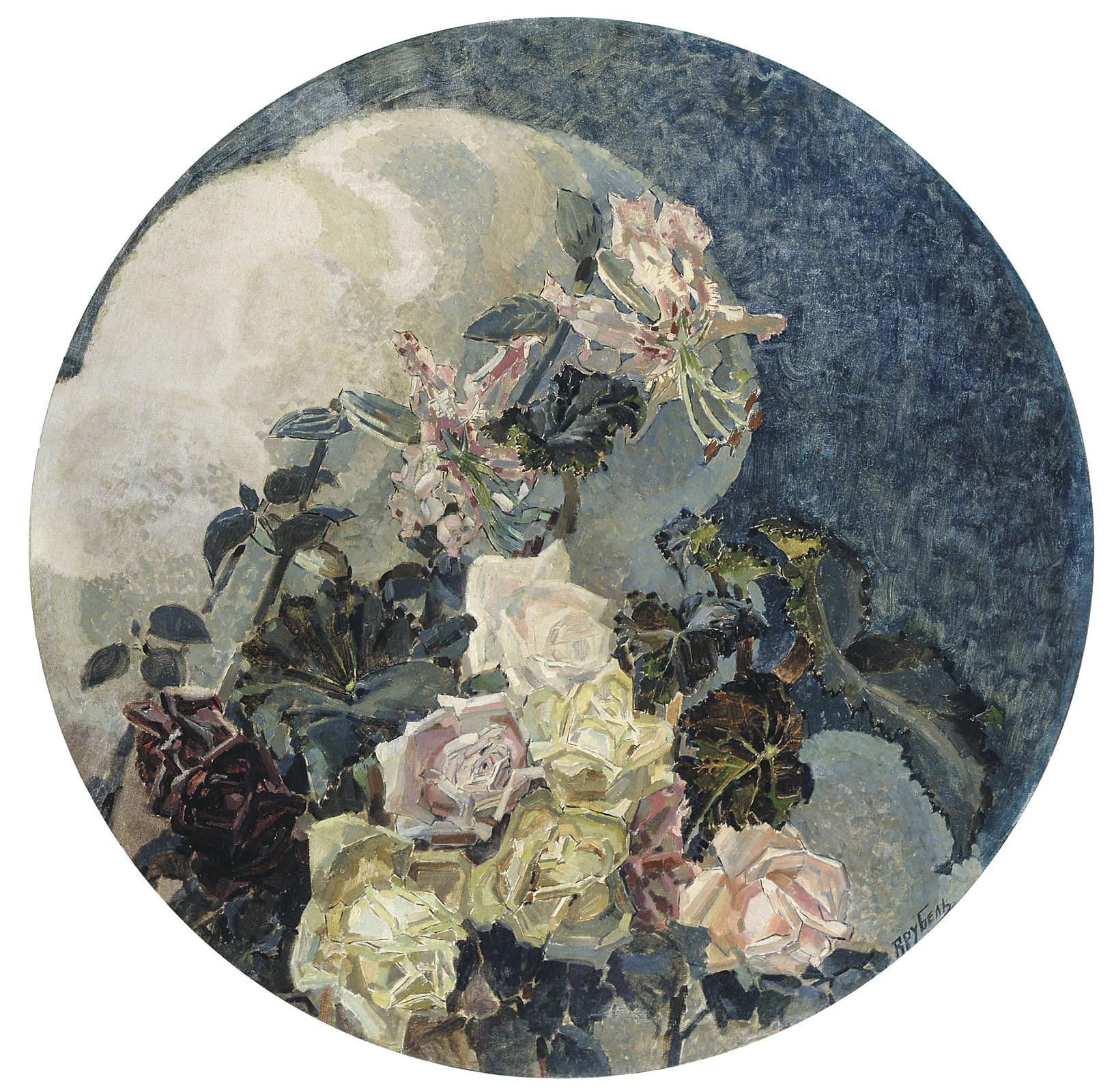The painting is a beautifully detailed, circular artwork featuring a vibrant floral arrangement set against a textured, bluish background. On the left side, there's a white, fluffy area, perhaps representing clouds. The central focus is a cluster of flowers and leaves, predominantly positioned towards the lower-middle section. The leaves blend seamlessly with the bluish background. The flowers include six roses of varying shades of pink and red, three in full bloom and three as buds, with thick, textured petals highlighted by visible brush strokes. In addition to the roses, there are four deep purple orchids with flared petals adding depth and variety to the arrangement. The contrast between the dark blue background and the vibrant, diverse flowers is striking, creating an image that's both dynamic and harmonious.